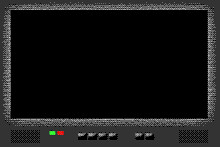An 8-bit graphic of a flat-screen TV with a grayish-black frame is prominently displayed. The TV features a large, darkened black screen that occupies nearly the entire frame. At the bottom of the frame, a series of controls and indicators are presented. From left to right, the layout includes a green light adjacent to a red light, followed by four buttons likely designated for power, volume, and channel functions. Further to the right, after a small gap, there are two additional black buttons. Flanking these controls on either side are two classic speakers, characterized by grid-like perforations, resembling the traditional design found at the bottom of vintage TVs.